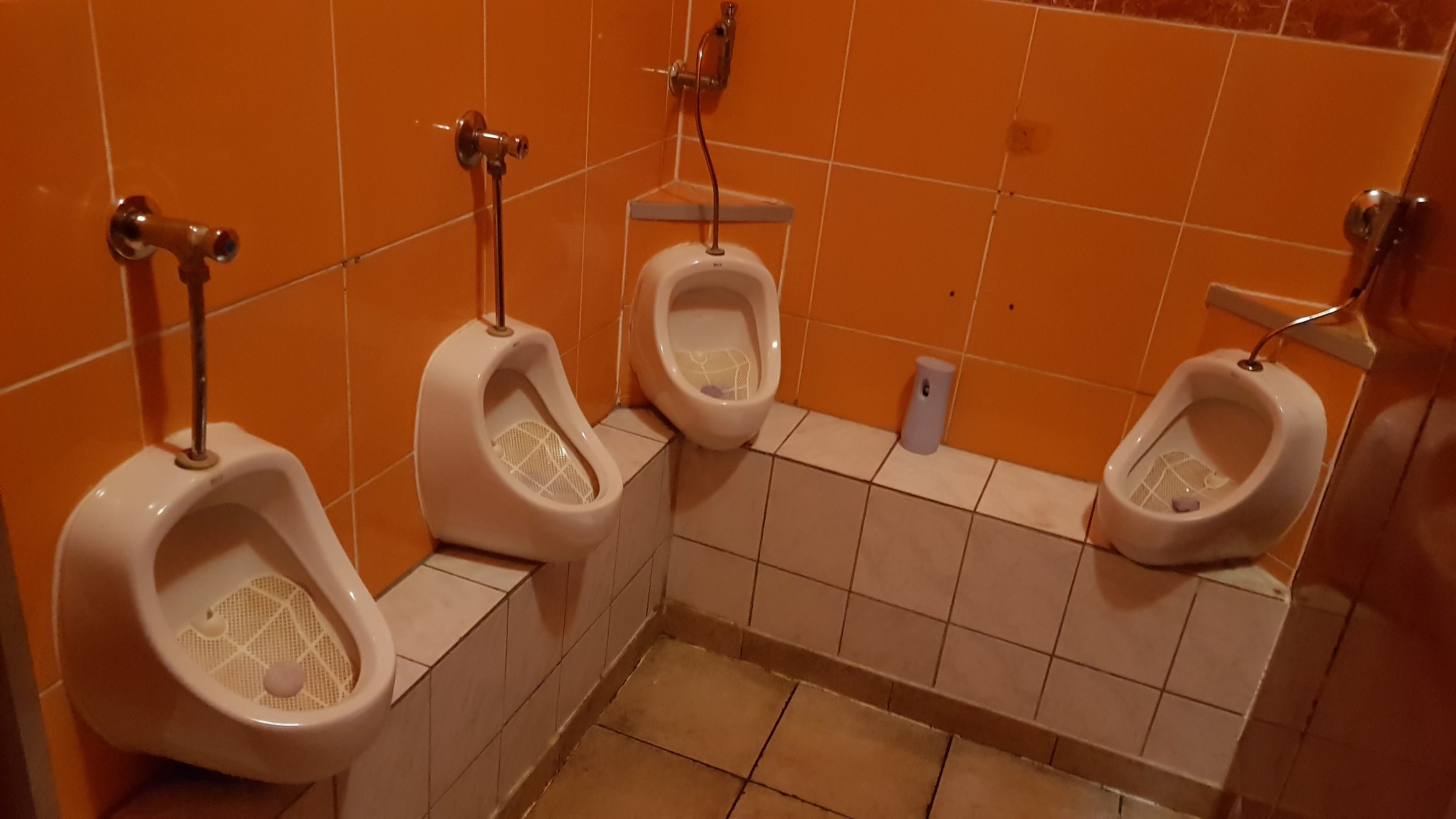This image is a photograph of the inside of a men's public restroom, oriented landscape-style. The restroom features four ceramic urinals with a short, stumpy design that extend outward and are mounted on a knee-high tiled ledge. The ledge, covered in white tiles, runs along the base of the urinals, providing a raised platform above the brown, somewhat discolored tile floor. The urinals are arranged uniquely: two are positioned on the left wall, one in the corner where two walls meet, and one on the adjacent wall, creating a compact setup with less than a foot of space between them. Metal pipes extend from the tops of the urinals, leading into the vibrant reddish-orange tiled walls. A gray automatic air freshener can be seen between two of the urinals. The restroom's wall tiles are divided into two sections: the lower half adorned with large orange tiles and the upper half with darker brown tiles, giving a distinct two-tone color scheme. The pipes and fixtures on the urinals are silver, adding to the industrial look of the restroom. Despite the tight space and obvious wear, the photo captures a unique and detailed view of a public bathroom's utilitarian design.